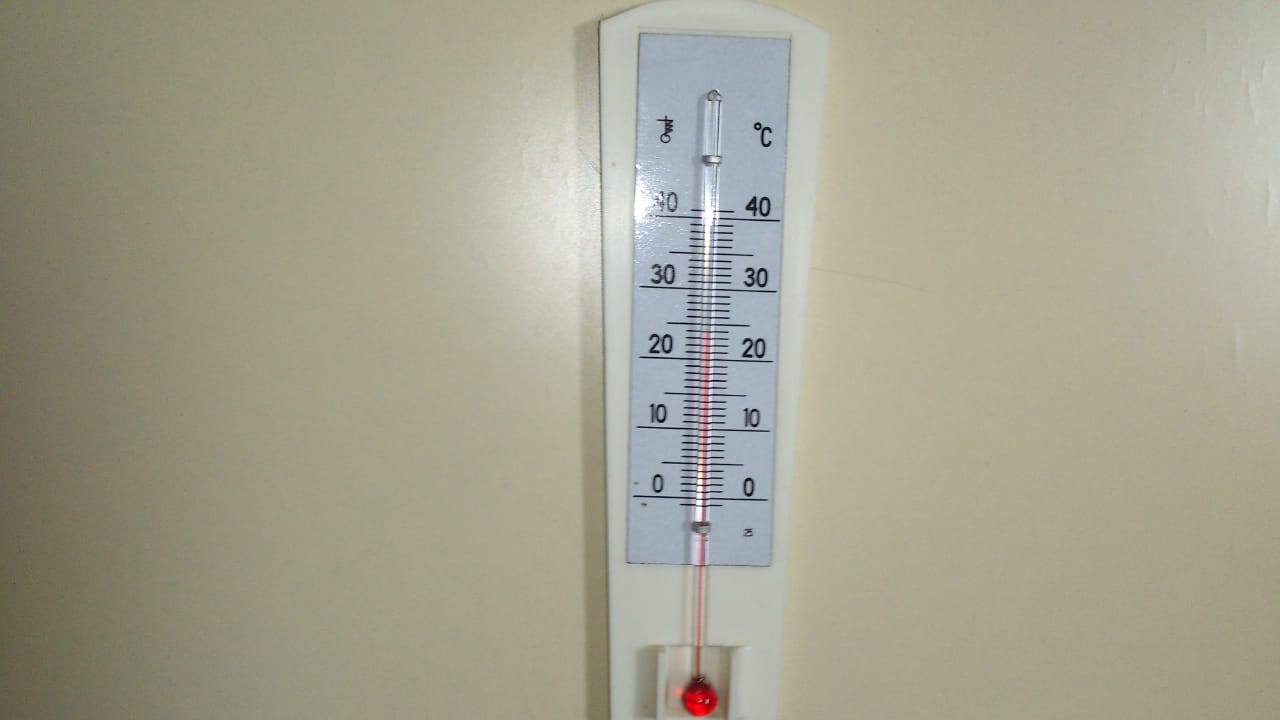This photograph showcases a white, wall-mounted analog thermometer composed of a snow-white plastic body. The temperature readings are centrally displayed in black font, etched onto a glossy white surface. A strip of glass runs through the center of the thermometer, containing a column of red liquid that indicates the temperature. On one side of the thermometer, there is a peculiar symbol resembling a cross with a circle and a squiggly line, while the other side displays a small circle and the letter "C." The temperature scale is marked in increments of 10 degrees, from 0 to 40. A camera flash is reflected off the glossy center of the thermometer, and the glass tube containing the red liquid is secured by two metal bands.